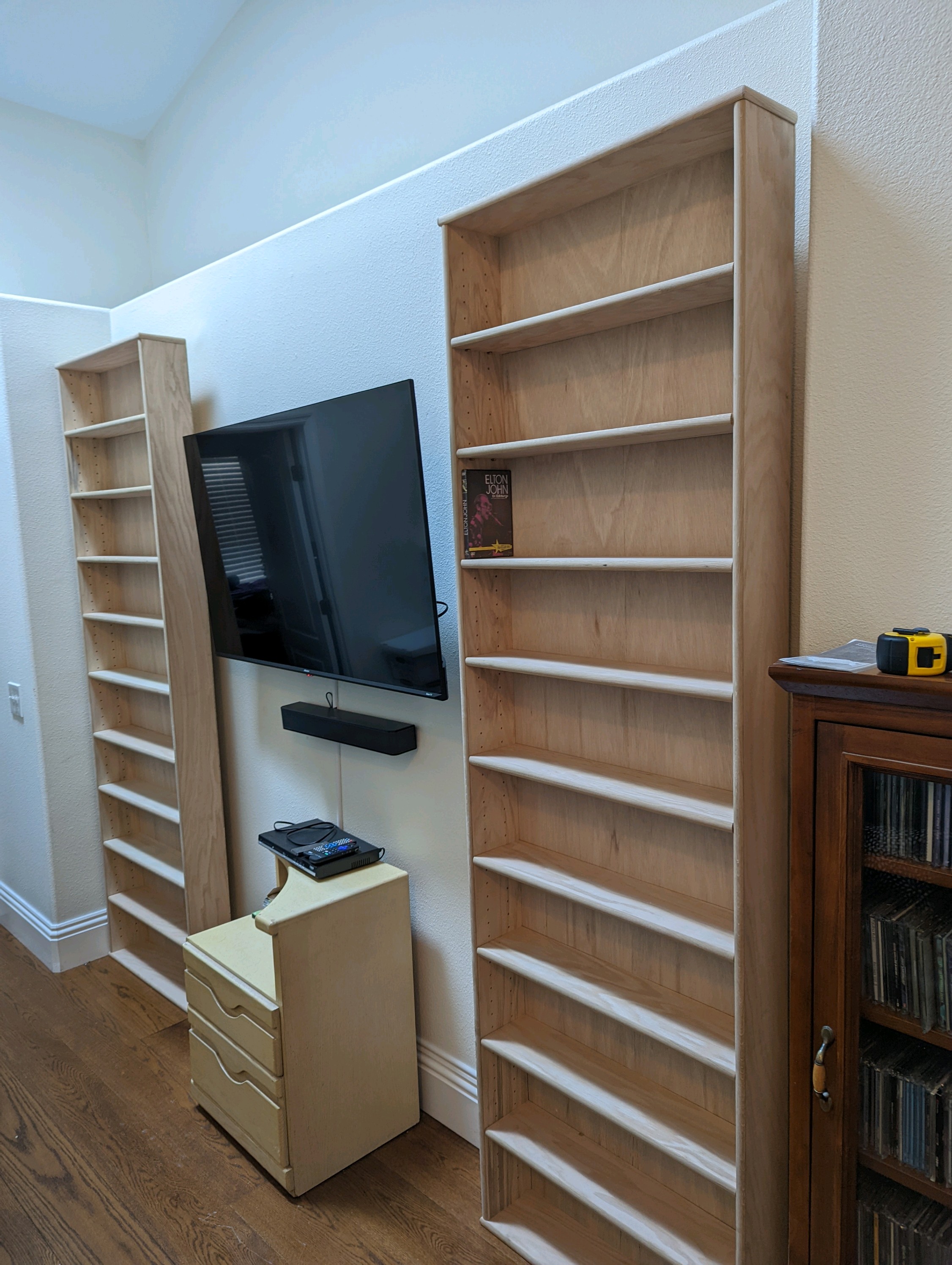The image captures a portion of a room with white walls, featuring a large flat-screen TV mounted on the wall with a sound bar directly below it. Below the TV, there's a small light tan wooden table, reminiscent of a nightstand, with two pull-out drawers. Sitting atop this table is a black Blu-ray or DVD player with visible cords. Flanking the TV are two very tall, narrow, medium-brown wooden bookshelves that extend almost to the ceiling. These shelves, interestingly, are predominantly empty, save for a solitary DVD—an Elton John movie. To the right, partially visible, is a dark brown cabinet with a glass door, which houses several CDs. The floor is finished with medium to dark brown hardwood tiles. The room’s layout is captured from a diagonal angle, providing a close-up of the right shelf and progressing towards the left where the smaller table and further shelf are located.